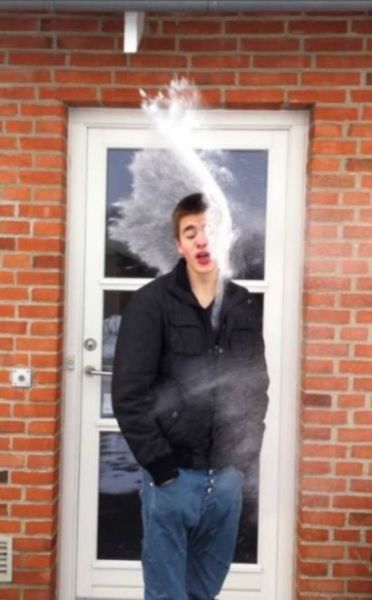In the surreal photograph, a young man stands with his eyes closed and mouth slightly open in front of a white glass-paneled gate of a brick building. He is dressed in a black jacket and blue jeans with his hands tucked into his pockets. An extraordinary splash of white fluid, possibly water, impacts the right side of his face, partially obscuring it and extending two to three feet above his head. This dramatic effect creates a striking visual element, giving an impression as if the fluid is either being forcefully shot at him or inexplicably emerging from his jacket.